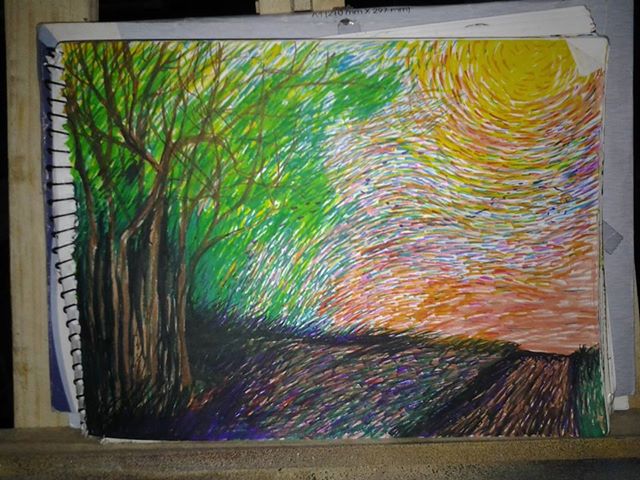This image is an intricately detailed illustration set in an outdoor environment, reminiscent of Van Gogh's "Starry Night" due to its heavily textured and hatched style. On the left side, brown-trunked trees stand tall with a canopy of vibrant green leaves stretching into the sky. The sun, positioned on the right side, is a brilliant yellow orb with dynamic lines radiating outward, transitioning from yellow to hues of red, purple, and a purplish-blue towards its center. Below the sun, the ground features a striking blue path that winds towards the trees. The base of the sketch integrates vivid tones, such as reddish-orange near the bottom right corner. The entire illustration is framed on what appears to be a sketchbook resting on a white surface, further supported by a wooden platform.